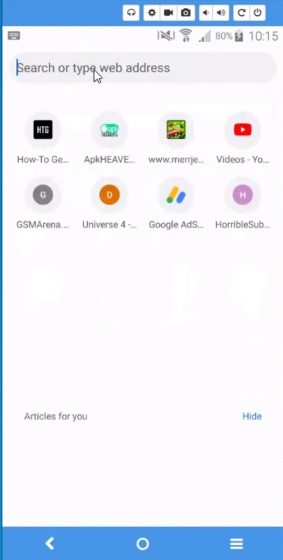The image captures a smartphone interface, showcasing various elements and functionalities. At the top row, the screen has a bluish tint, flanked on the right side by several icons that serve as navigation buttons, directing users to different sections. Below this, there are several status symbols indicating the phone's various settings, such as vibration mode, signal strength, battery level, and the current time. Further down, there's a prominent search bar labeled "Search or type web address," designed for web searches and URL entries.

Continuing down, more icons are visible, which are shortcuts to frequently used apps like YouTube and other miscellaneous applications. At the very bottom of the screen, there are three primary navigation buttons: a back button, a home button, and a multitasking button that allows the user to switch between open windows. Additionally, there's an option to hide certain elements, and below the main navigation, there's a space reserved for more articles or suggested content for the user.